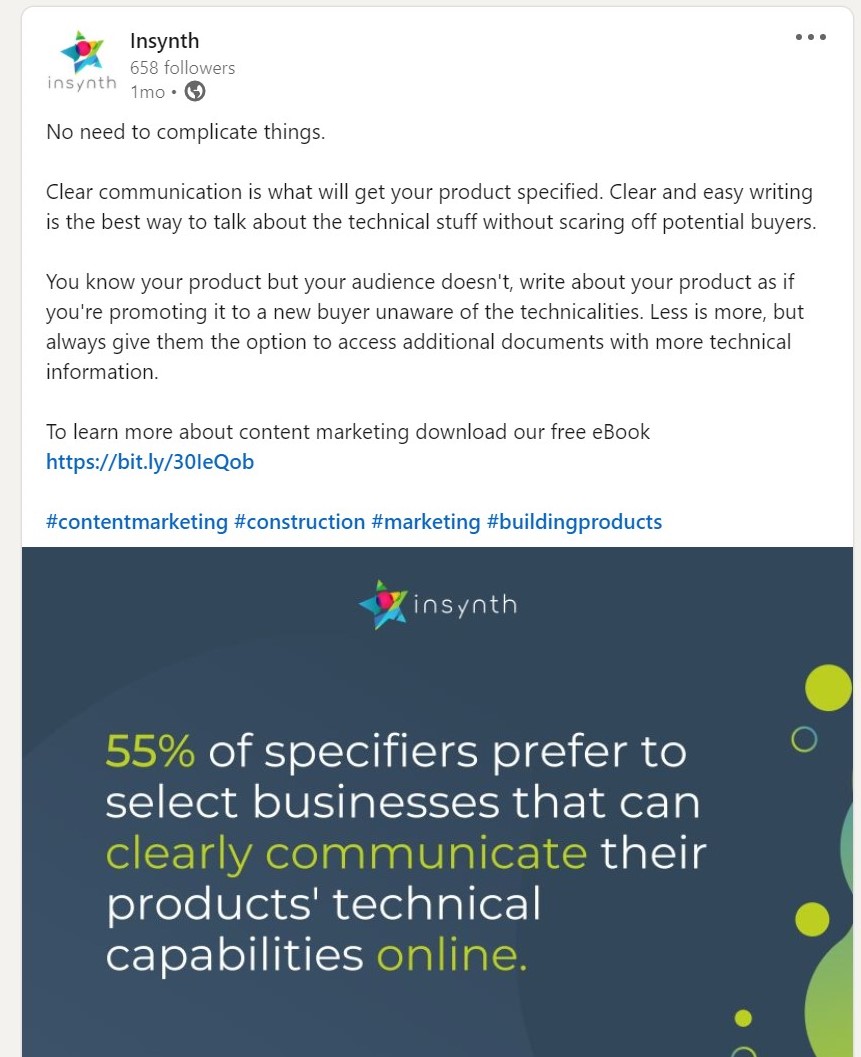Below is a detailed and cleaned-up caption for the provided image description:

---

**Screenshot of a Social Media Post by InSight**

InSight, boasting 658 followers, shared a post one month ago emphasizing the importance of simplicity in communication. The post reads:

"No need to complicate things. Clear communication is what will get your product specified. Clear and easy writing is the best way to talk about the technical stuff without scaring off potential buyers. You know your product, but your audience doesn't. Write about your product as if you're promoting it to a new buyer, unaware of the technicalities. Less is more, but always give them the option to access additional documents with more technical information. To learn more about content marketing or to download our free e-book, visit [URL]."

The post is accompanied by the hashtags: #contentmarketing, #construction, #marketing, #buildingproducts.

**Visual Description:**

- **Graphic:** The InSight logo features a star and is set against a dark blue background with green accents. 
- **Statistic:** A prominent stat highlights that "55% of specifiers prefer to select businesses that can clearly communicate their products' technical capabilities online." The words "55%", "clearly communicate," and "online" are highlighted in green.
- **Additional Design Elements:** Green circles appear to the right of the frame, adding a visual accent. 
- **Interface:** The ellipsis (three dots) in the top right-hand corner suggests additional settings or sharing options.

This post by InSight underscores the necessity of clear and concise communication in effectively marketing technical products, without overwhelming potential buyers.